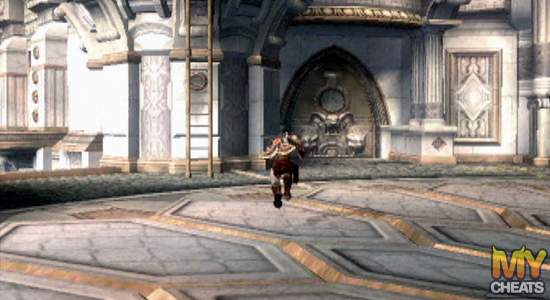This detailed screenshot from the video game "God of War" features the iconic character, Kratos, centrally positioned and seemingly running towards a ladder within an opulent, ancient setting. Kratos is depicted from behind, adorned in battle gear and wearing brown boots. The scene is set on an intricately designed platform or floor, showcasing an off-white octagonal pattern with gold trimming. The surrounding environment resembles a grand, Greek-inspired architectural structure, detailed with exquisite carvings, columns, and archways. The background includes stonish walls, varying between gray and white with elaborate designs, possibly indicating a castle or palace. Additionally, there's a notable bull's head with large horns framed within a pointed archway, which might symbolize a clock or an emblematic feature. In the bottom right corner of the screenshot, the text "My Cheats," with the "M" displaying small devil horns, suggests it might be a watermark from a gaming magazine or website.